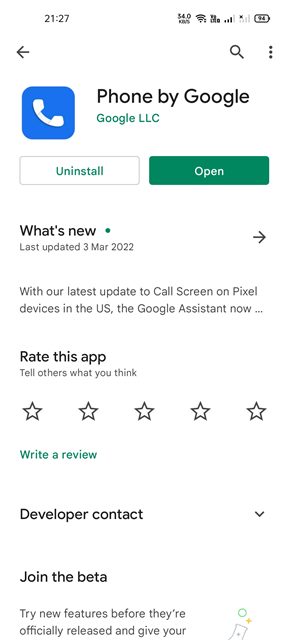**Detailed Caption:**

The image showcases a Google Play Store screen displaying the installation page for the "Phone by Google" app, which is the default phone application for Android devices. The screen highlights the app name "Phone by Google" along with the developer's name. Users are presented with options to either uninstall or open the app. Additional details include the app's last update date, which is listed as March 3, 2022. Further user interactions are available, such as rating the app, writing a review, contacting the developer, and an option to join the beta testing program, which is intriguing for a phone application. At the top of the screen, standard mobile interface elements are visible, including a device icon, a search bar, and a three-dot menu for additional functions.

Overall, the layout and elements are what one would expect from a Google Play Store app listing, making it clear that this is indeed the installation screen for the "Phone by Google" app.